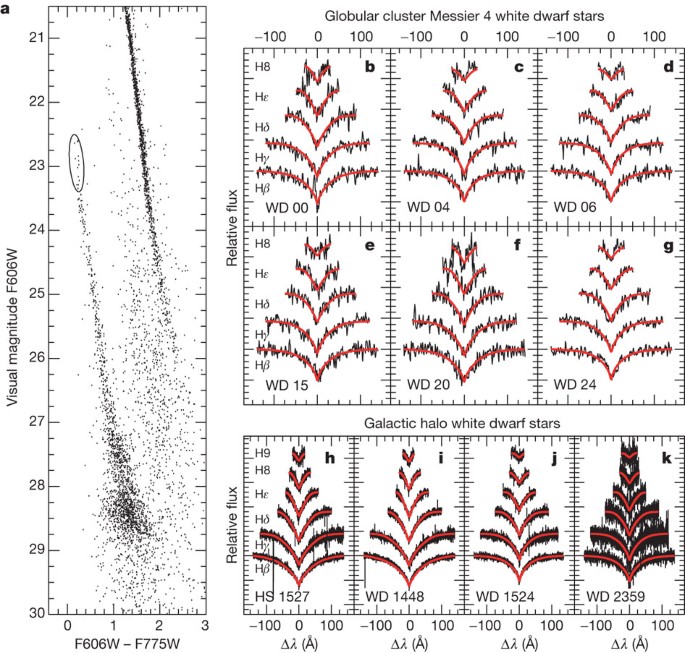This detailed image showcases stellar datasets and analyses. Dominating the left side is a scatter plot chart labeled "Visual Magnitude (F606W)" on the vertical axis and "F606W - F775W" on the horizontal axis, which features markings from 0 to 3 in incremental hash marks and a vertical range of 21 to 30. The scatter plot reveals dense concentrations of data points around specific coordinates, notably near (1.5, 28.5) and toward the upper section around (1.75, 21-22). 

The top right portion displays six detailed sub-boxes, organized in two rows of three, titled "Globular Cluster Messier 4 White Dwarf Stars," containing individual graphs with axes labeled "Relative Flux" (vertical) and "WD" (horizontal). At the bottom right, another set of detailed graphs is labeled "Galactic Halo White Dwarf Stars." The entire image is filled with red lines and dots arranged in a complex, tree-like pattern, suggesting an intricate network of stellar data visualizations emphasizing white dwarf stars within different cosmic structures.